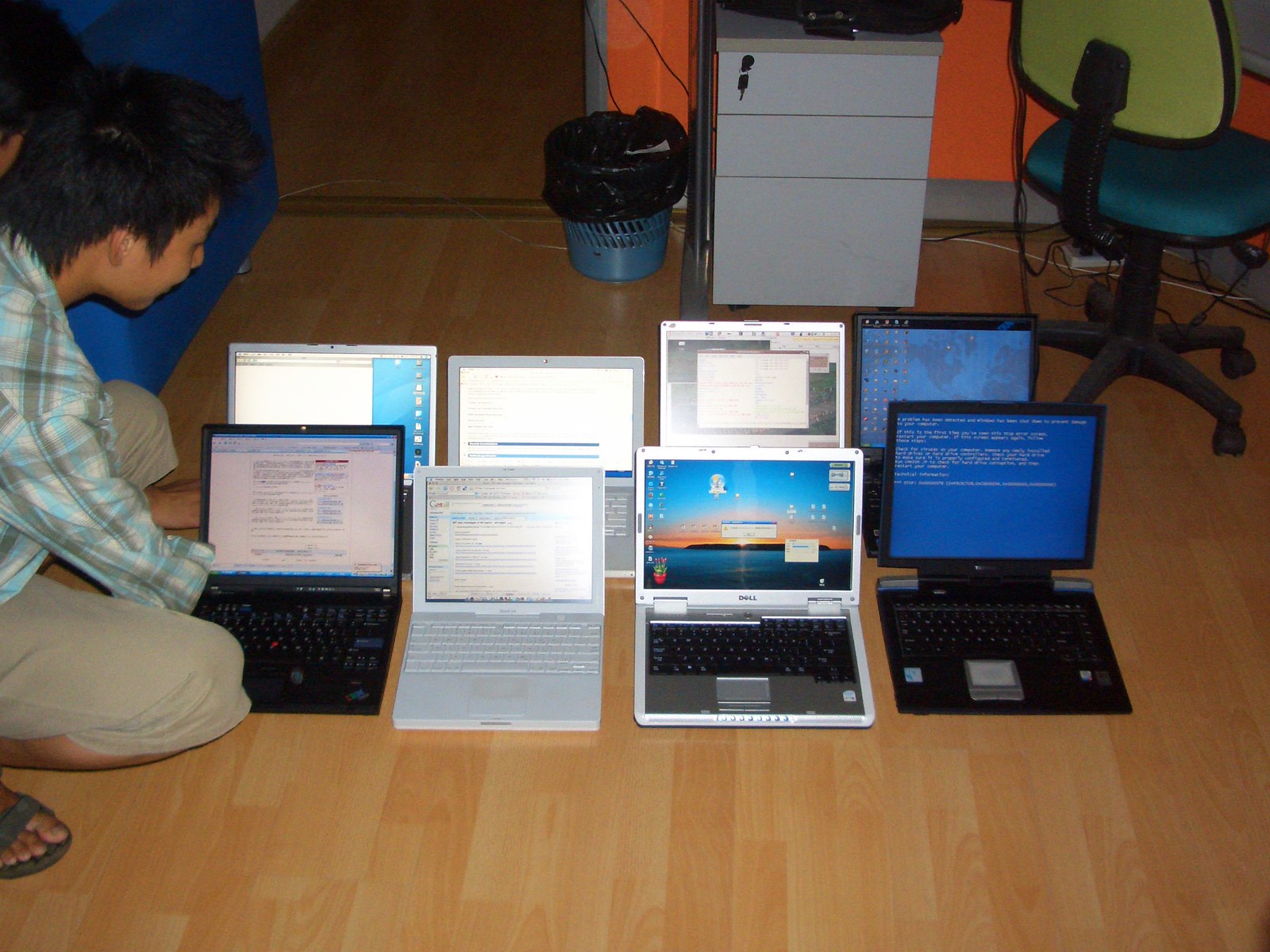The image captures a detailed interior scene, likely a dorm room or study area, showcasing eight different models and brands of laptop computers arranged on a tan brown wooden floor. The laptops are organized in two rows of four, each screen displaying various outputs such as spreadsheets, dialog boxes, or the infamous blue screen of death. In the midst of this technical array, a man with short spiky black hair is kneeling on the left side of the photograph. He is donned in knee-length khaki pants and a plaid shirt in shades of blue, white, and gray. Behind him, the room extends into a hallway, evidenced by an open door and a glimpse of the hallway floor. Adjacent to the door is a small wastebasket with a black liner, and nearby stands a grayish-beige file cabinet. A notable green-backed, aqua blue-cushioned rolling office chair sits to the right, complementing the room's practical, yet busy atmosphere. The man, intently observing the varied states of the laptops, appears focused and possibly troubleshooting the array of devices before him.